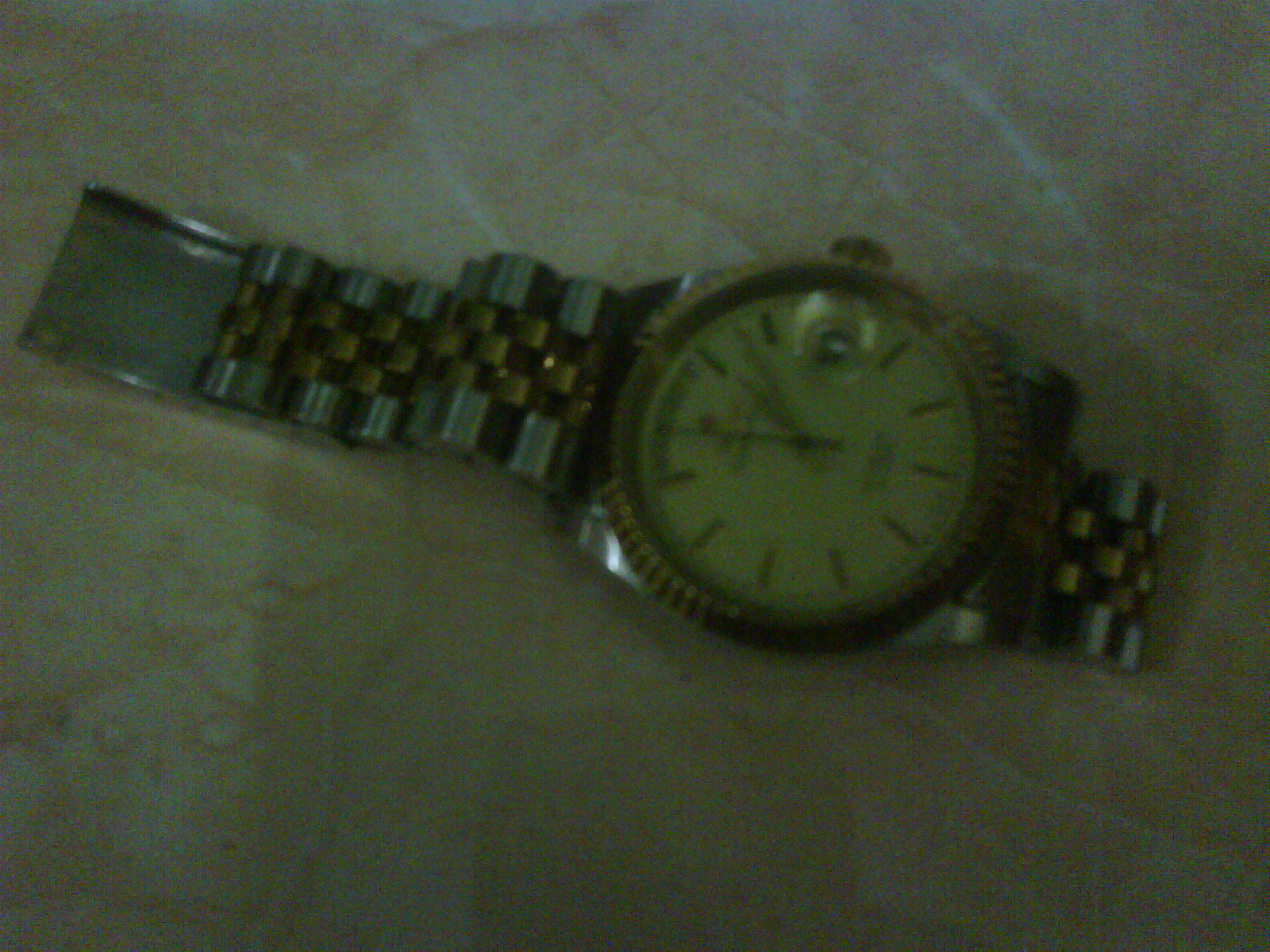The image captures a somewhat dim and slightly blurry close-up of a wristwatch placed horizontally on a marble or granite countertop. The band features a blend of silver and gold, with the central part of the band displaying gold links amidst larger silver ones. The watch face, positioned slightly to the right of the center, has a clean white background adorned with gold lines and no numerical markings. The hands indicate it's nearly ten past one. A date dial with a magnifier peeks out from the watch face. The countertop beneath showcases a mix of white to cream to orangey shades, adding a warm, textured backdrop to the composition. Despite the low resolution, the intricate details of the watch and the nuanced tones of the countertop are discernible, albeit mildly obscured by the darkness and blurriness of the photo.